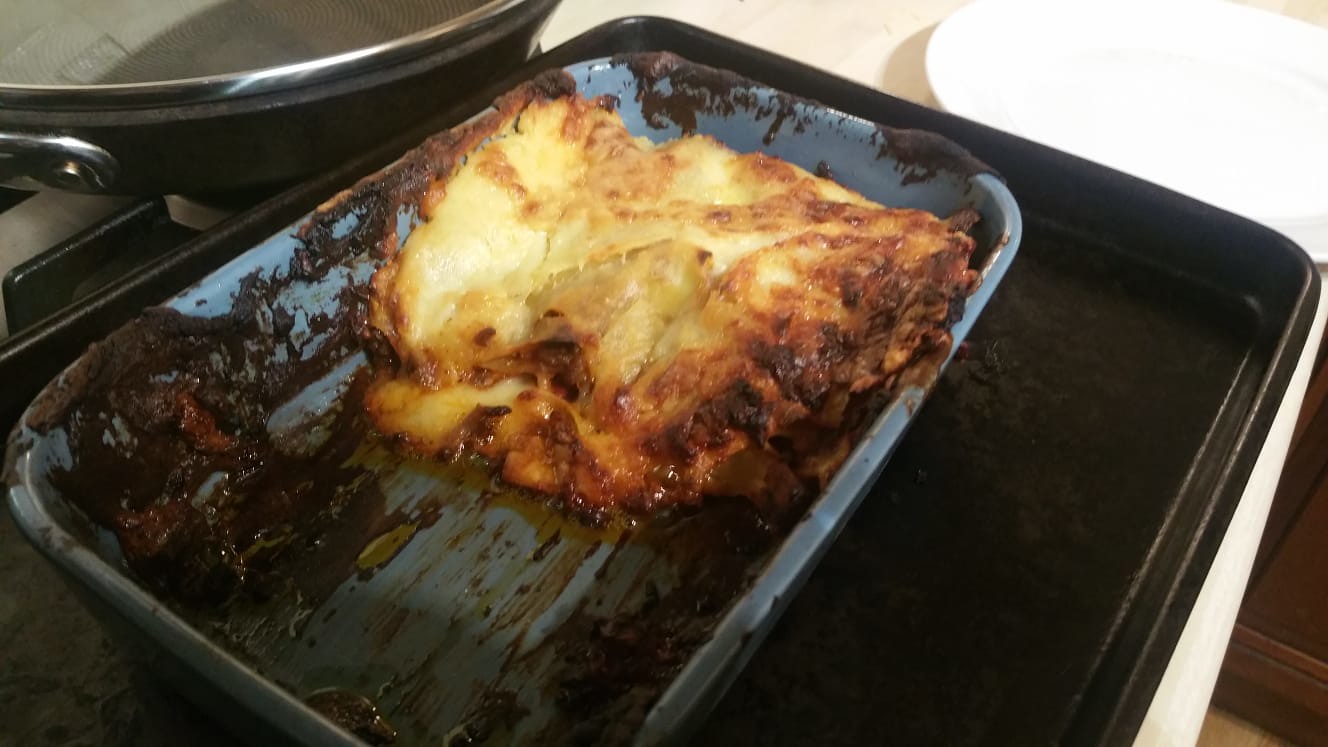The image depicts a cluttered kitchen countertop featuring a prominently placed light blue rectangular baking pan containing roughly 40% of a lasagna. The lasagna, with its layers of tomatoes, cheese, and pasta noodles, is angled towards one o'clock and sits atop a larger, darker baking sheet that shows signs of extensive use with baked-on residues. The edges of the lasagna are noticeably burnt, displaying dark brown to almost black scorch marks. The countertop itself appears to be black, though one description mentions a white counter. In the upper left-hand corner of the image, there is a black pan with silver lateral striping and a lid, while an empty white plate occupies the upper right-hand corner. The overall scene suggests a recently used kitchen space with remnants of a meal still visible.